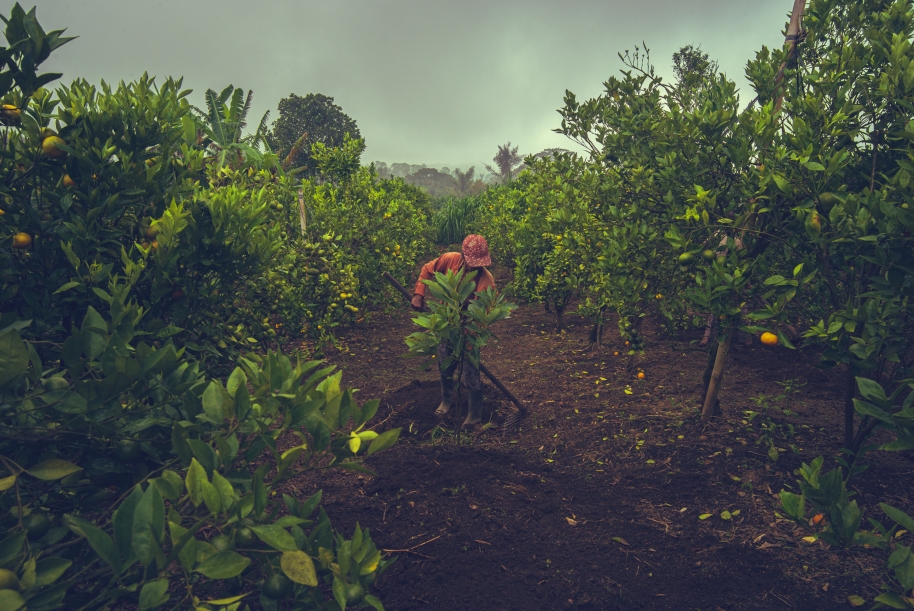The photograph captures a farmer, whose gender is indistinguishable, amidst an expansive orange grove, marked by dense rows of green-leaved trees extending into the horizon. The image is framed from within one of the dirt rows, featuring lines of fruit-bearing trees on either side, laden with unripe orange fruit. At the center, the farmer, dressed in an orange long-sleeved shirt, an orange hat or ball cap, dark colored pants, and black boots, is working diligently. The individual holds a hoe and appears to be planting a small fruit tree, notably shorter and smaller than the surrounding mature trees — the young tree only reaches their shoulder height. The farmer is in the process of cultivating the black soil around this new sapling, carefully raking the earth to ensure the roots are covered. The gray sky in the backdrop enhances the greenery of the grove, encapsulating the scene of agricultural labor.